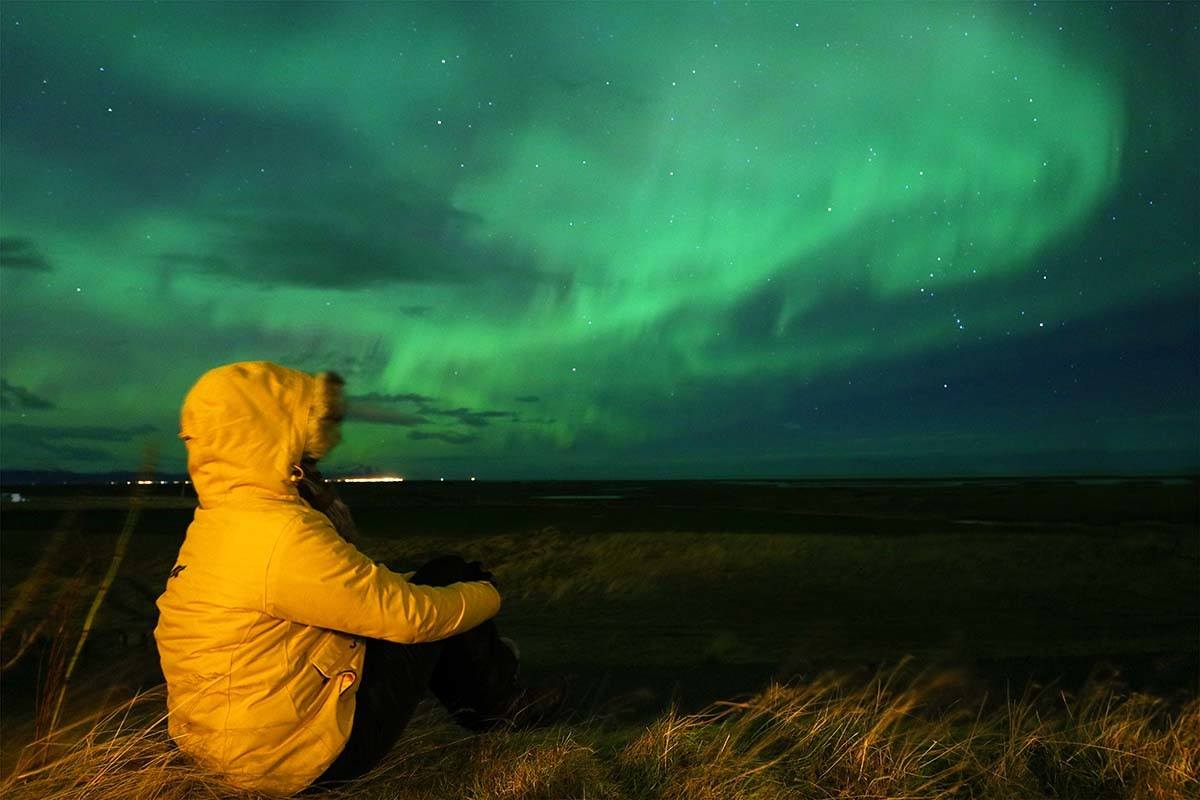The photograph captures a person seated on the tall, windswept grass, looking skyward on a dark night. The individual is wearing a hooded yellow parka and black pants, with their back to the camera, making it difficult to discern their gender. They seem mesmerized by the brilliant display of the aurora borealis, with swirling sheets of green interspersed with a variety of colors lighting up the sky. The background reveals a clear night filled with stars, including the recognizable outline of the Orion constellation. In the distance, faint lights—likely from buildings or a harbor—dot the horizon, suggesting the person has ventured far from the city's illumination to better witness the natural phenomenon. The scene exudes a cold, windy atmosphere, with the tall grass bending under the gusts. The night sky, adorned with the mesmerizing northern lights and twinkling stars, stands as the true centerpiece of this serene and mystical setting.